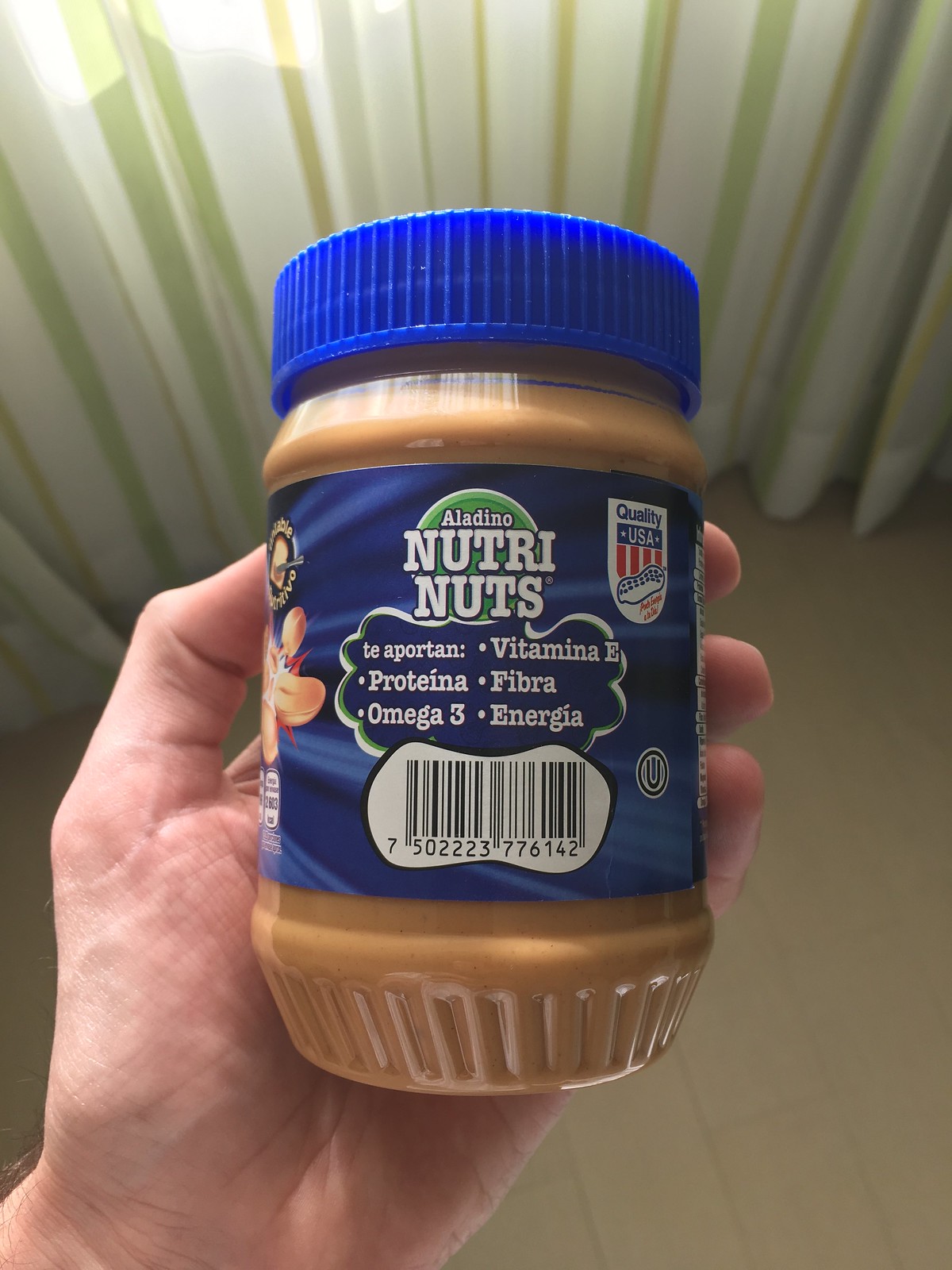This photograph features a man's left hand holding a jar of Aladino Nutri Nuts peanut butter. The hand, with its fingers curled around the jar, has a visible thumb on the left and three fingers on the right. The jar itself is round with a royal blue screw-on lid, and a darker blue label wrapping around it. The label prominently displays the brand "Aladino Nutri Nuts" in white text, along with nutritional highlights in Spanish: "Vitamina E," "Proteína," "Fibra," "Omega-3," and "Energía." On the upper right of the label, there is a red, white, and blue shield emblem marked "Quality USA." Also featured on the label is a white bubble containing a barcode shaped like a peanut. The background of the image consists of light brown or pale green tile-like flooring, transitioning to a plastic curtain adorned with alternating stripes of white, green, and gold.